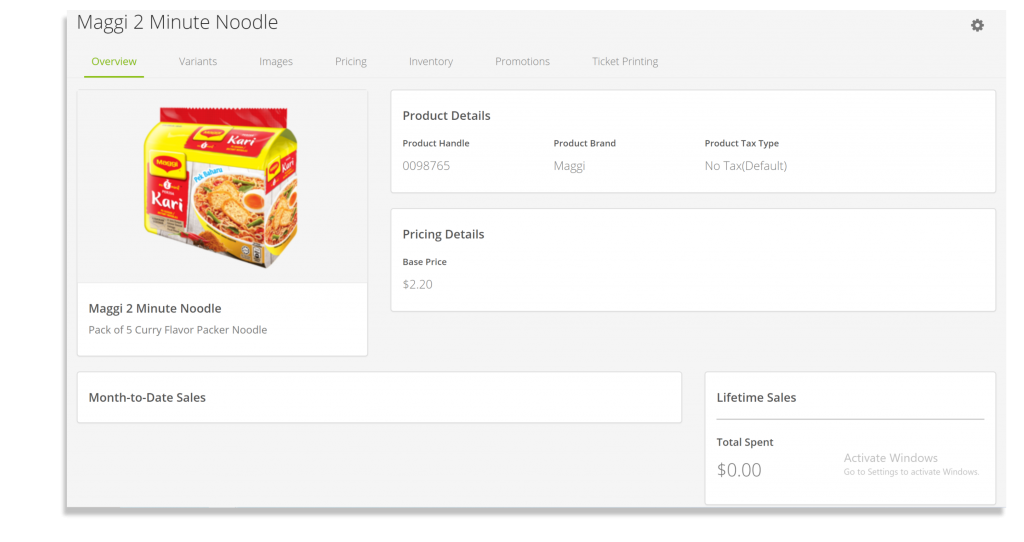**Descriptive Caption:**

This image showcases a detailed screenshot of a website interface, likely an e-commerce product management page. The layout features a gray background at the top left-hand corner and prominently displays the "MAGGI Two Minute Noodle" brand. A navigation menu is present, with the active page displayed in underlined green text. The other menu items are in gray text and include options such as Variants, Images, Pricing, Inventory, Promotions, and Ticket Printing. 

At the top right corner, there is a gray settings icon. On the left-hand side of the screen, a visual image of the product is depicted, showing a yellow and red pack of noodles with an illustration of a bowl of ramen. Below the image, the product is labeled as "MAGGI Two Minute Noodle pack of five, curry flavor." 

Under this label, there is a white box titled "Month Date Sales." On the right-hand section of the interface, a separate white box displays product details in black text, listing: Product Handle 0098765, Product Brand MAGGI, and Product Tax Type: No Tax (default). 

Further down, another identically shaped white box outlines the pricing details: the base price of the item is $2.20. Finally, at the bottom right-hand corner of the image, a small white box titled "Lifetime Sales" is shown, indicating that the total spent is $0.00. Additionally, a notification at the bottom right mentions "Activate Windows - Go to Settings to activate Windows."